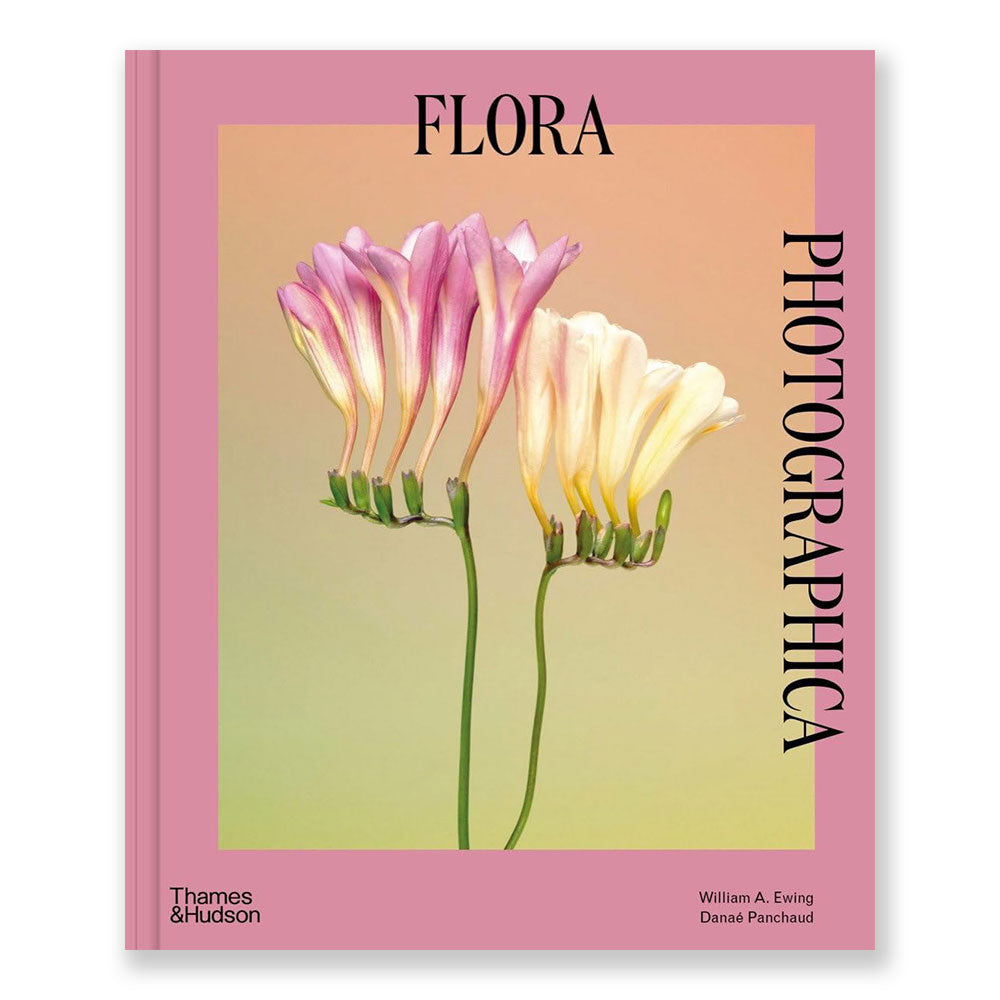The cover of the book "FLORA" features bold black capital letters at the top with the word "Photographica" written vertically on the right side. The central image showcases elegant plant life with pink and yellow-white flowers on delicate, wiry green stems. The flowers on the left side are a rich pink, taller with some green buds, while the right side displays slightly shorter yellow-white flowers. The background transitions from a peach color at the top to a lime green at the bottom. A light pinkish-purple border frames the cover, thicker on the sides and bottom. The bottom left corner bears the name of the publisher, Thames and Hudson, while the bottom right corner lists the authors or photographers, William A. Ewing and Denae Penchode, in sans serif font.